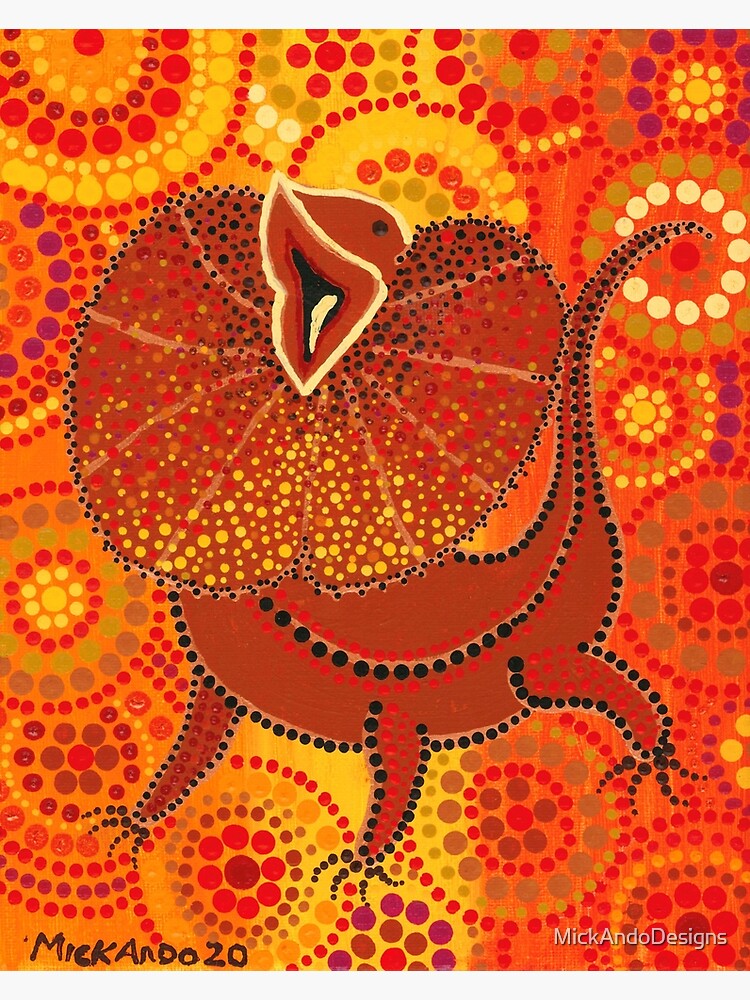The image showcases a vibrant, stylized painting of a frilled lizard with an abstract twist. This distinctive artwork, credited to McAndo Designs, features the lizard with an open mouth and a fan-like frill spreading from the lower jaw, reminiscent of a Venus flytrap. The creature is detailed with black eyes and claws, a long whippy tail, and red and black dotted patterns. Its head and mouth are highlighted with yellow outlines. The intricate background is a mosaic of circular patterns in various hues, including red, orange, green, and yellow. Notably, the painting has watermarks on both corners; the one on the bottom left is seamlessly painted as "McAndo Designs," whereas the one on the bottom right appears digitally overlaid.